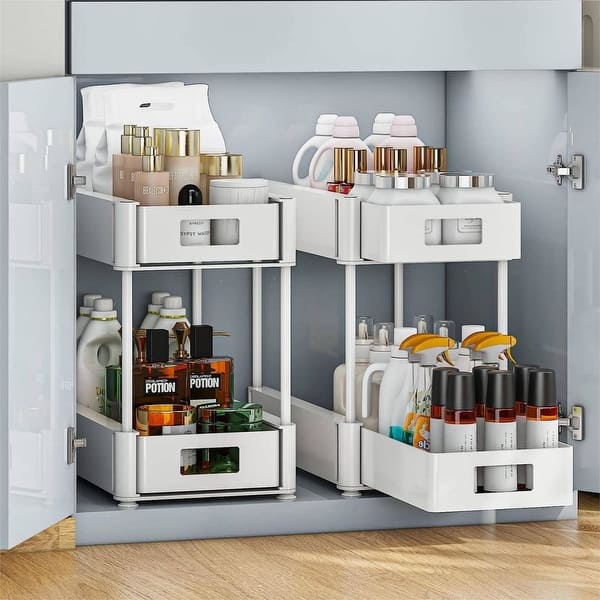This indoor photograph showcases an open cabinet, likely situated beneath a bathroom sink, accentuated by its soft, pale blue color. The cabinet doors, affixed with metal hinges, are swung open to reveal two white shelves within. Each shelf features pull-out drawers, organized with numerous bottles and containers. The top drawers predominantly contain makeup products, including candles, soaps, and perfumes, with bottles labeled "potion" and possibly laundry detergent. The lower drawers house more utilitarian items such as pump bottles and spray bottles, suggesting an assortment of cleaning supplies and personal care products. Notably, the highly reflective cabinet surface mirrors the stored items. The entire setup rests on a wooden floor, enhancing the sense of a well-organized, functional space in what is likely a bathroom.